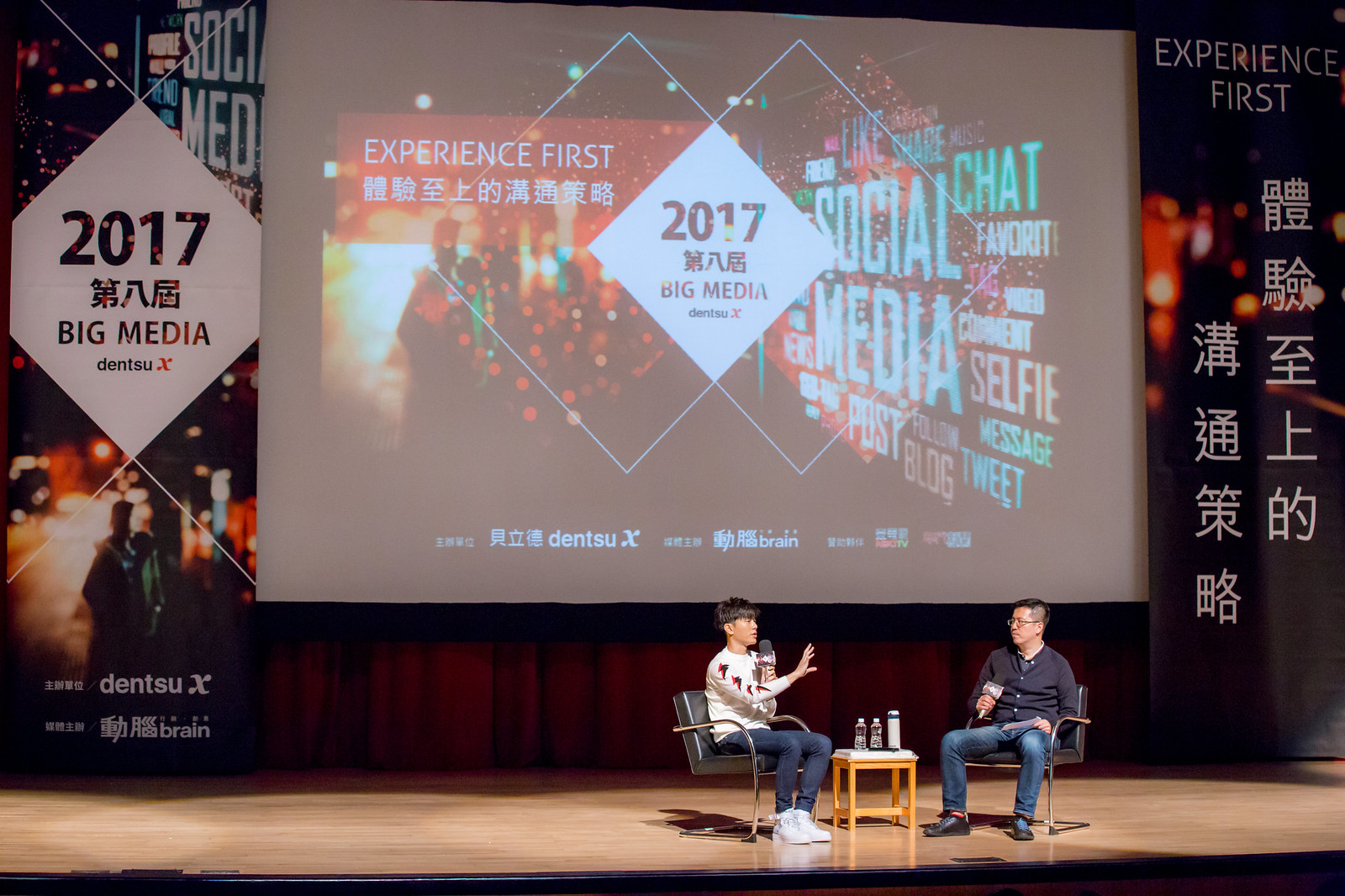This indoor photograph captures the vibrant atmosphere of a significant convention held in Japan in 2017, aptly named the "2017 Big Media Meeting." Central to the image are two Asian gentlemen positioned on a lit stage, seated in utilitarian yet comfortable black chairs. A small, square wooden table between them holds a few bottles of water. Each man clutches a microphone, with the gentleman on the left currently speaking. The man on the left is dressed in a white shirt and jeans, while his counterpart on the right wears a dark blue, possibly black, button-up shirt.

Behind them, a pull-down screen prominently displays a slightly washed-out projection reading "2017 Big Media Experience First," surrounded by a collage of social media buzzwords like "social media," "chat," "selfie," and "tweet." Enhancing the backdrop, banners adorned with vertical Japanese characters and photographs showcasing Japan flank the screen on either side, adding cultural depth to the event's setting. The image encapsulates a moment of dialogue and engagement at a media-focused gathering.